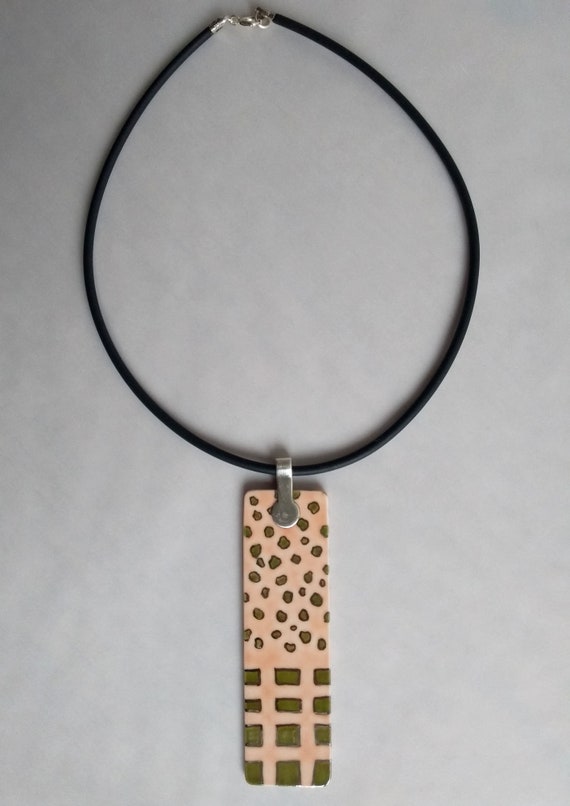The image showcases an abstract piece of jewelry, possibly a choker necklace, presented in a top-down photograph on a light blue to slate gray background. The centerpiece of this necklace is a rectangular pendant with a pink Himalayan sea salt hue. The top half of the pendant features an arrangement of small brown or bronze circular stones, while the bottom third consists of twelve small squares in the same brown or bronze color, resembling an African-inspired design. This pendant is connected to a black loop—likely leather or string—via a silver metal clasp at the top. The entire composition is set against a minimalistic backdrop devoid of distinguishing features.